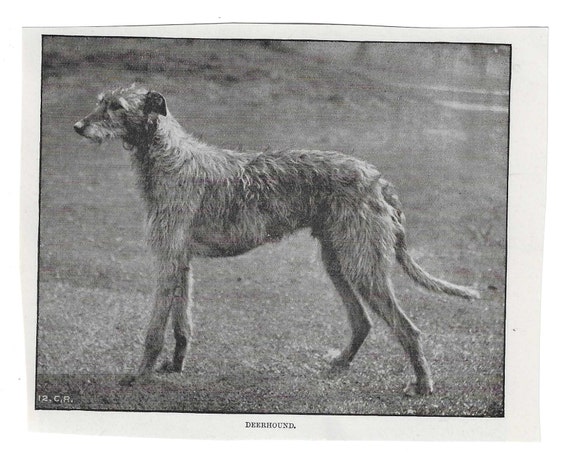The vintage black and white photograph depicts a tall, average-sized dog with scruffy, curly hair, standing in a grassy field. The dog, identified as a deerhound in a caption at the bottom of the image, has shorter but shaggy fur, particularly around its mouth. It has short ears that perk up slightly and a long tail. The dog appears somewhat unkempt, with fur that looks matted and dirty, displaying a mottled color of dark brown and dirty white. The photo, which seems to have been clipped from a newspaper or book, features an uneven white border around it and a slight black border within. In the lower left corner, there's a marking indicating "12.C.R." The dog gazes towards the left side of the image with a sense of alertness, as if listening for something in the distance. The background hints at a low hill and a row of houses in the upper right corner.